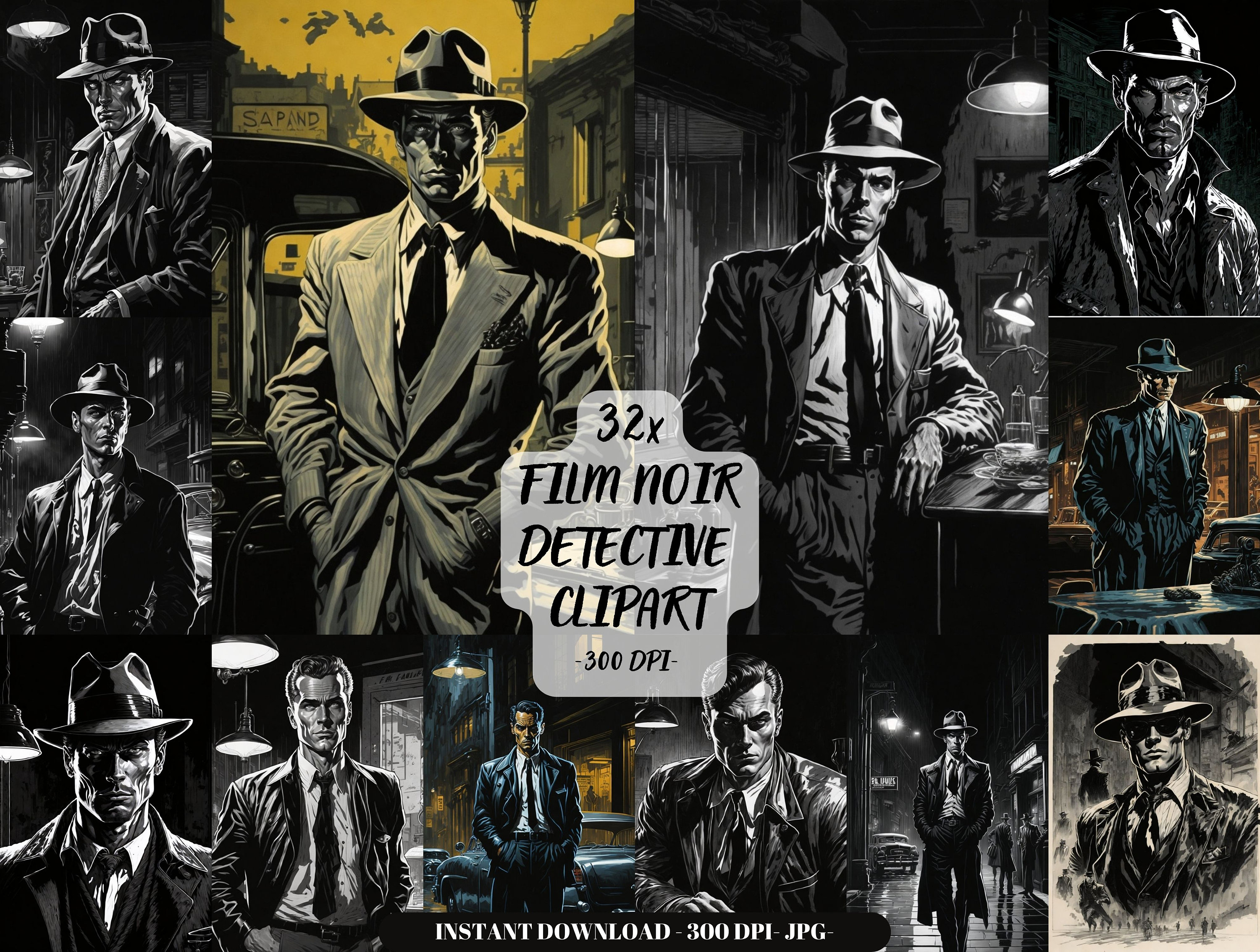The image is a meticulously crafted poster or collage featuring twelve or so film noir detectives in various poses, predominantly in black and white with occasional yellow hues. Each detective exudes a serious demeanor, characteristic of the film noir genre, and they are uniformly dressed in classic 1950s detective attire: hats, suits, ties, and in some cases, leather jackets or trench coats. The layout is a landscape format, presenting these detectives in close-up shots, mostly from the waist, chest, or leg up, capturing their stern expressions in dimly-lit settings reminiscent of bars or street corners.

In the center of the image, bold text reads "32x Film Noir Detective Clip Art 300 DPI" against a white-gray background, emphasizing the comprehensive collection of detective imagery. The poster also features a larger image in the upper left corner with a yellow background, highlighting a detective in a brown suit. The bottom of the image reinforces its digital utility with the text "Instant Download 300 DPI JPEG" in white.